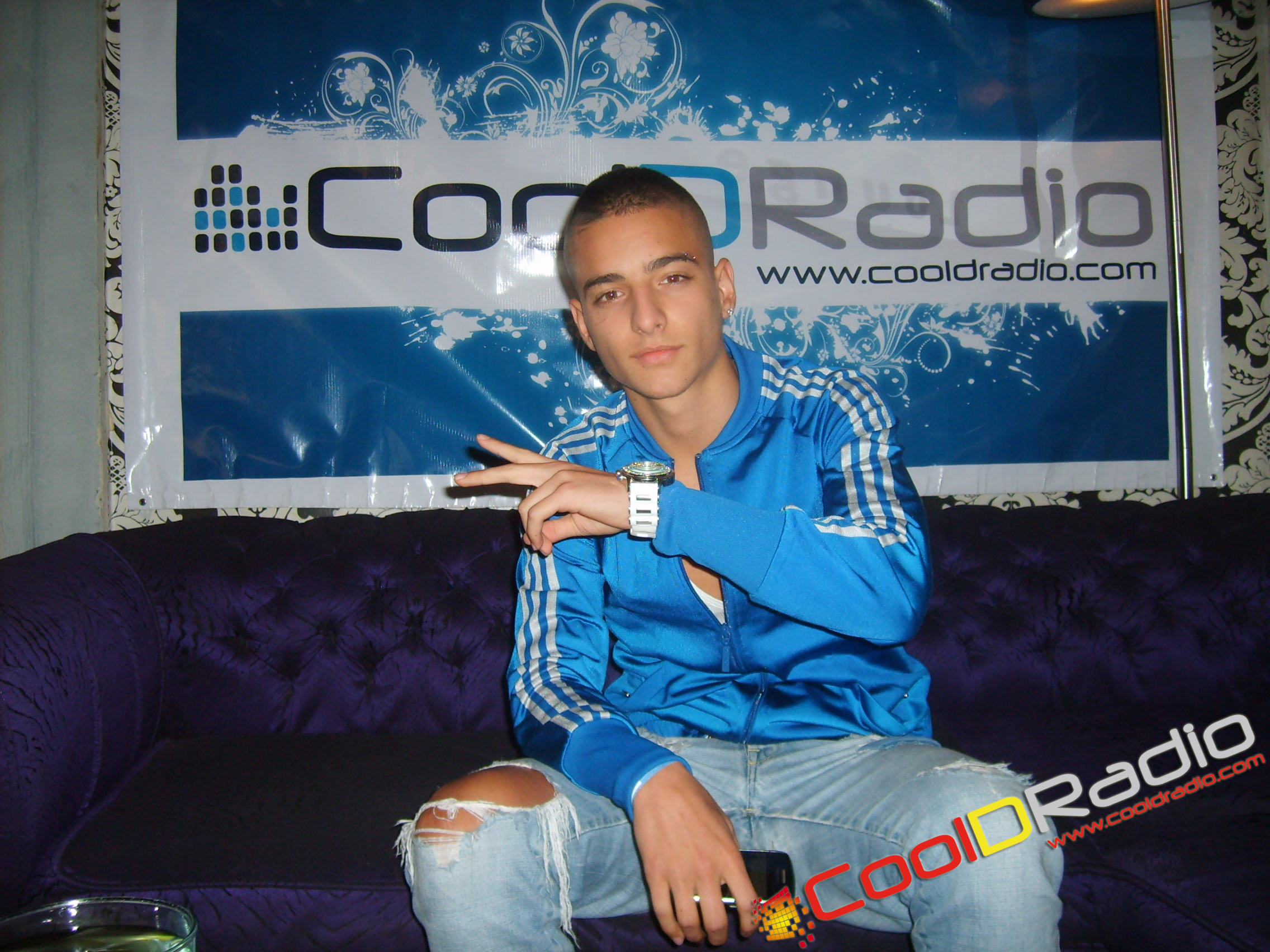This detailed color photograph captures a young, possibly white or Middle Eastern male seated on a plush dark bluish-purple couch. The man, who could be a DJ or an enthusiast of Cool D Radio, is dressed in a light blue Adidas track jacket adorned with white stripes on the sleeves. Beneath his jacket, which is left open, a glimpse of a white T-shirt is visible. He pairs this with light blue, distressed jeans that feature a tear on the left leg and a significant rip exposing his right knee.

His appearance is marked by a very short, close-shaven haircut, particularly trimmed along the edges, brown eyebrows, and brown eyes. His expression suggests a closed-mouth smile. On his left wrist, he sports a large watch with a white band.

The backdrop features an eye-catching advertisement for Cool D Radio. Dominating the wall behind him is a large blue banner with a white border. The banner prominently displays the text "Cool D Radio" and the website "www.cooldradio.com," with the "D" text placed in light blue between the words "Cool" and "Radio." Additional decorative elements on the banner include a swirling, almost floral-like white pattern against the blue background. The young man's head slightly obscures part of this banner. In the lower right corner, the banner includes another "Cool D Radio" inscription in red, yellow, and white, along with a website listing in red letters.

In this horizontal photograph, estimated to be around 8 by 7 inches, the composition includes his right hand resting on his knee, potentially holding a cellphone, and his left hand extended across his chest, forming a peace sign. This visually descriptive image effectively melds personal style with promotional messaging for Cool D Radio.